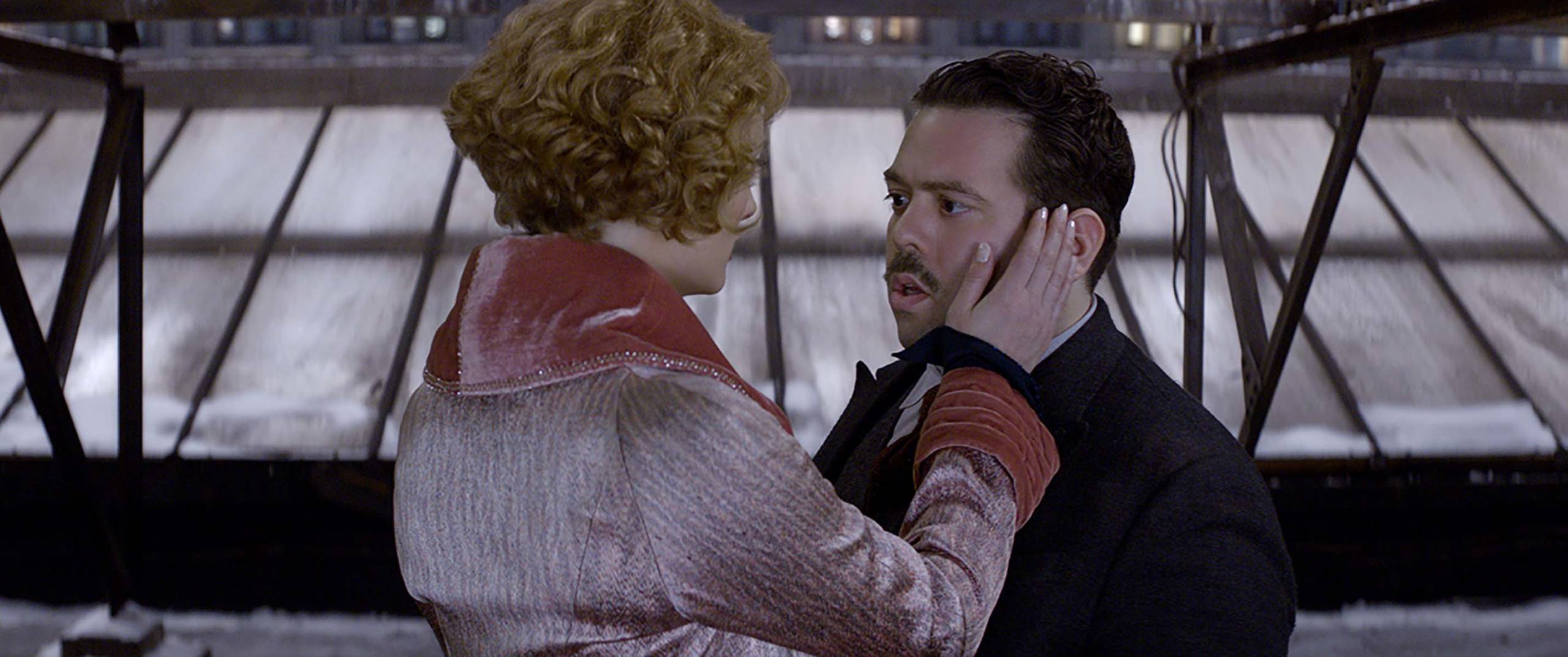The image appears to be a cinematic still from a movie, possibly associated with the Harry Potter series. It captures a poignant moment between a man and a woman, framed in a panoramic shot that suggests a rooftop setting against a backdrop of buildings with lit and unlit windows. Dominating the background is a large, spherical glass structure with black borders, punctuated by platforms, railings, and supporting legs. 

At the center of this scene stands the couple, engaged in an intimate gaze. The woman, with short, curly brown hair styled in a vintage fashion, is dressed in a distinctive coat. Her coat features a striking large red leather collar and wide red sleeves, with the rest of the garment being a muted pink adorned with subtle patterns. She gently places her right hand on the man's cheek, her eyes locked onto his, conveying a sense of comfort or consolation.

The man, who has neatly combed black hair and a small mustache, appears unsettled. His eyes, possibly brown, are cast downward, and his lips are parted as if he is speaking. He is clad in a black suit over a white shirt and overall presents a slightly disheveled appearance. The scene is framed in a way that enhances the emotional tension between the characters, set against the architectural details and the ambient light of the surrounding cityscape.